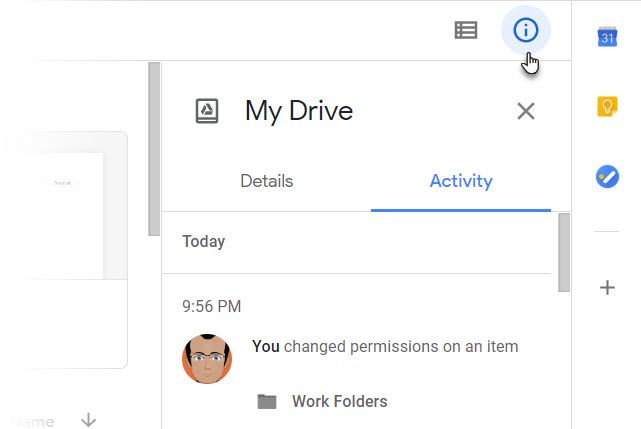This caption describes a detailed screenshot of a Google Drive web page with specific elements highlighted. Below is the cleaned-up and detailed description:

---

This image is a detailed screenshot of a Google Drive web page. The background is white with a very thin horizontal gray line across the top. The image appears to be scrolled toward the right side, as the left part is cropped off. On the left side of the image, there is a vertical scroll bar that can be dragged up and down, though its specific purpose is not clear.

At the top-right corner of the page, there's a menu icon followed by a pale blue circle with a dark blue 'i' inside, serving as an information button. An outlined hand icon with a pointing finger indicates the information button.

On the right side of the page is a column featuring several icons: a calendar icon, an icon that might be related to 'About' (shown as a light bulb on a yellow square), and another icon that could possibly be for editing.

The main section of the screen displays the heading "My Drive," next to which is a logo reminiscent of a recycling symbol, formed by chasing arrows. There is also an 'X' button next to "My Drive" to close it.

Beneath the main header are two tabs: "Details" and "Activity." Currently, "Activity" is selected and highlighted in blue with a blue underline, while "Details" remains grayed out. Below the active "Activity" tab is a white bar with the label "Today," separated by a thin gray line leading to the activity details.

The activity log shows an entry at 9:56 PM stating, "You changed permissions on an item," with "You" in bold. There is also an avatar of a male with dark hair and glasses indicating the user. The item affected is identified as "Work folders," accompanied by a folder icon.

---